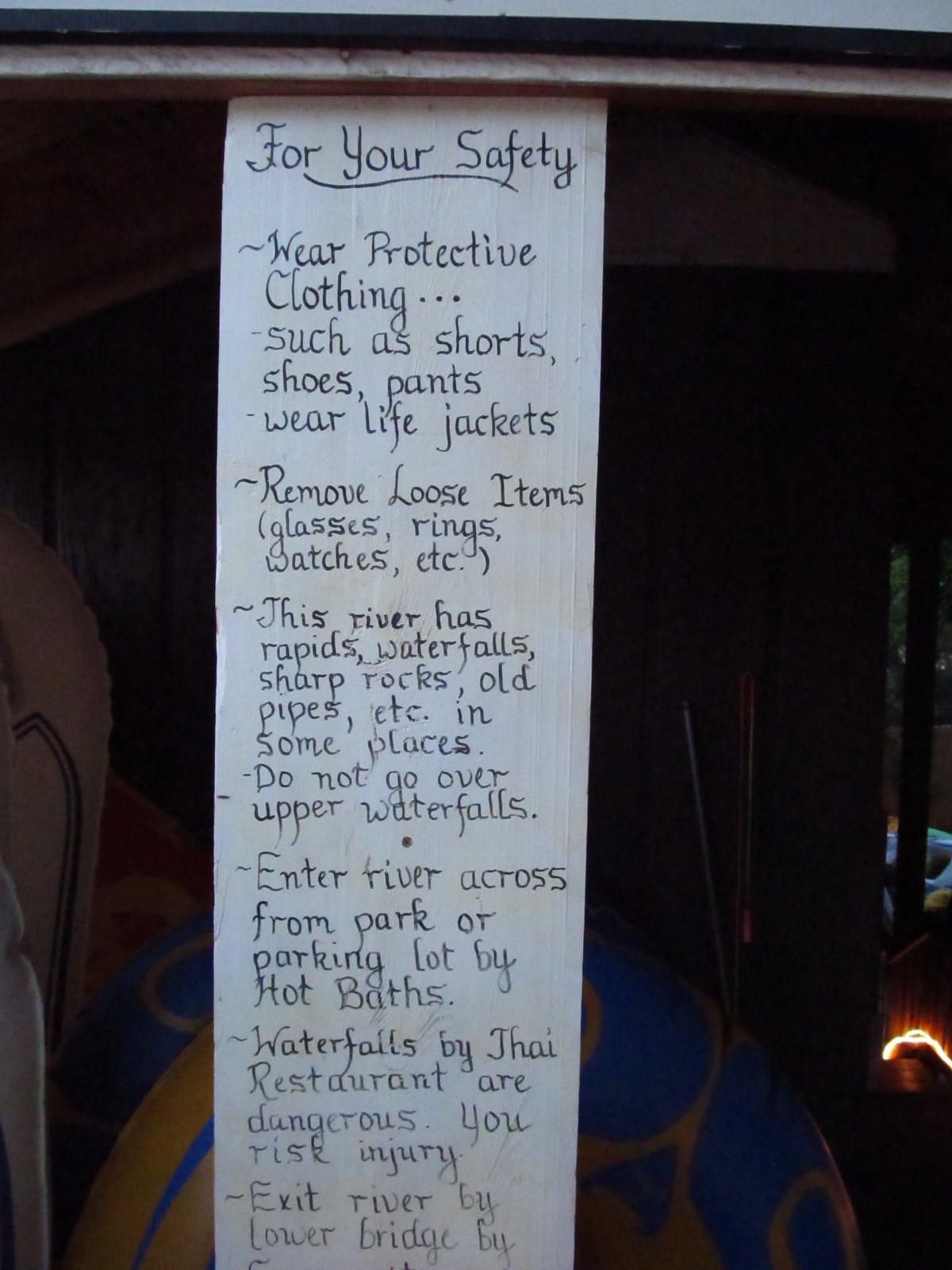The image features a large handwritten sign with black text on a white sheet of paper, suspended from a pipe against a dark background. The sign, detailed and neatly written, includes important safety instructions for navigating a hazardous river area. It advises wearing protective clothing such as shorts, shoes, and life jackets, and removing loose items like glasses, rings, and watches. The text warns about the presence of rapids, waterfalls, sharp rocks, and old pipes in the river. It specifically cautions against going over the upper waterfalls, advises entering the river across from the park or parking lot by the hot baths, and highlights the danger of waterfalls near a Thai restaurant. It instructs to exit the river by a tower near the lower bridge. A slight illumination from a neon light is visible in the lower right corner, adding a subtle glow to the scene.